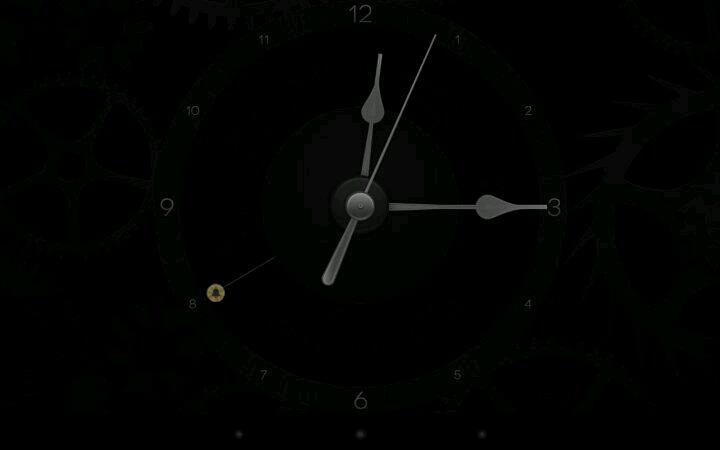In the image, a clock is partially visible, shrouded in darkness which makes it challenging to discern its features. Despite the low light, a faint hint of green emerges from the clock's design. The numbers, subtly highlighted in gray, follow the standard sequence from one to twelve in a clockwise manner. The clock is equipped with three hands—minute, hour, and second—each in gray. An additional instrument featuring a gold circle at its end points toward the eight, adding an unusual detail to the clock's appearance. Surrounding the periphery of the clock is a green pattern, possibly depicting wheels or a unique design element. In the inlay of the clock, a green representation of Earth is visible, enhancing its distinctiveness. The time displayed by the clock reads approximately 12:15.